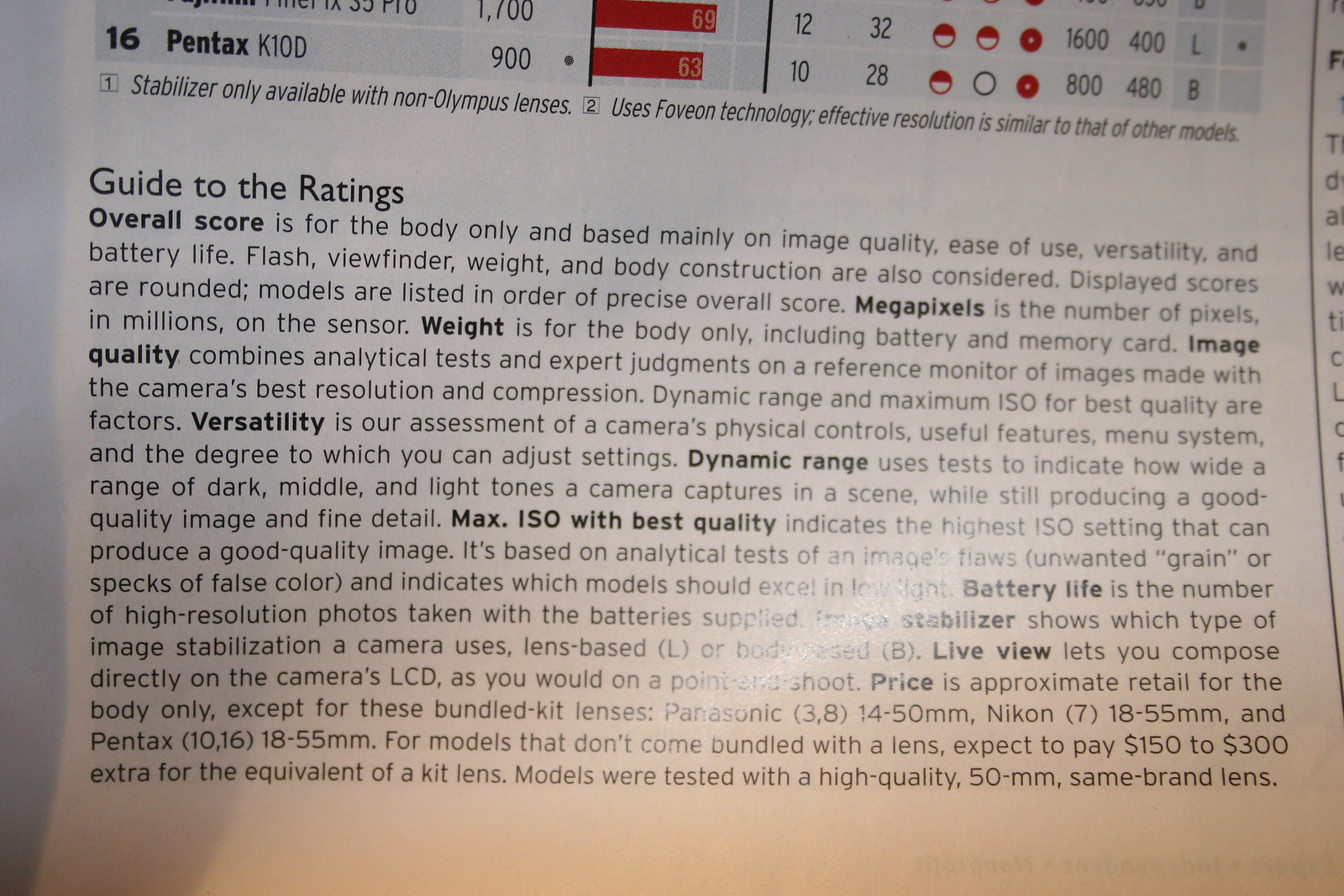The image appears to be a photograph of a screen or a printed page, with a slight reflection visible in the bottom right corner. The background is white, and the text, formatted in black, spans from the top left to the bottom right. At the top of the image, the title "Guide to the Ratings" is prominently displayed. The text is segmented and includes several bolded terms: overall score, megapixels, weight, image quality, versatility, dynamic range, max ISO with best quality, battery life, stabilizer, live view, and price.

The article outlines the criteria used for evaluating camera models. The overall score, focused solely on the camera body, is derived mainly from image quality, ease of use, versatility, and battery life, though factors like flash, viewfinder, weight, and body construction are also considered. Scores are rounded, and models are listed by their precise overall scores.

Megapixels refer to the millions of pixels on the sensor. The weight mentioned includes the camera body, battery, and memory card. Image quality is assessed through a combination of analytical tests and expert judgment on a reference monitor, considering aspects like resolution and compression, dynamic range, and maximum ISO for best quality.

Versatility evaluates the camera’s physical controls, useful features, menu systems, and the extent to which settings can be adjusted. Dynamic range tests determine how well a camera captures dark, middle, and light tones while maintaining fine image details. Max ISO with best quality identifies the highest ISO setting that can still produce top-quality images, focusing on analytical results about flaws, such as unwanted grain or false color specks, to highlight models excelling in low light.

Battery life is quantified by the number of high-resolution photos taken with the supplied battery. Stabilizer information indicates the type of image stabilization used, whether lens-based or body-based. The live view function allows composing images directly on the camera’s LCD, similar to using a point-and-shoot camera.

Prices quoted are approximate retail values for the camera body only, except for specific bundled kit lenses from Panasonic (38, 14-50mm), Nikon (7, 18-55mm), and Pentax (10-16, 18-55mm). For models without bundled lenses, an additional $150-$300 may be required for a kit lens equivalent. The models were tested using high-quality 50mm lenses from the same brand.